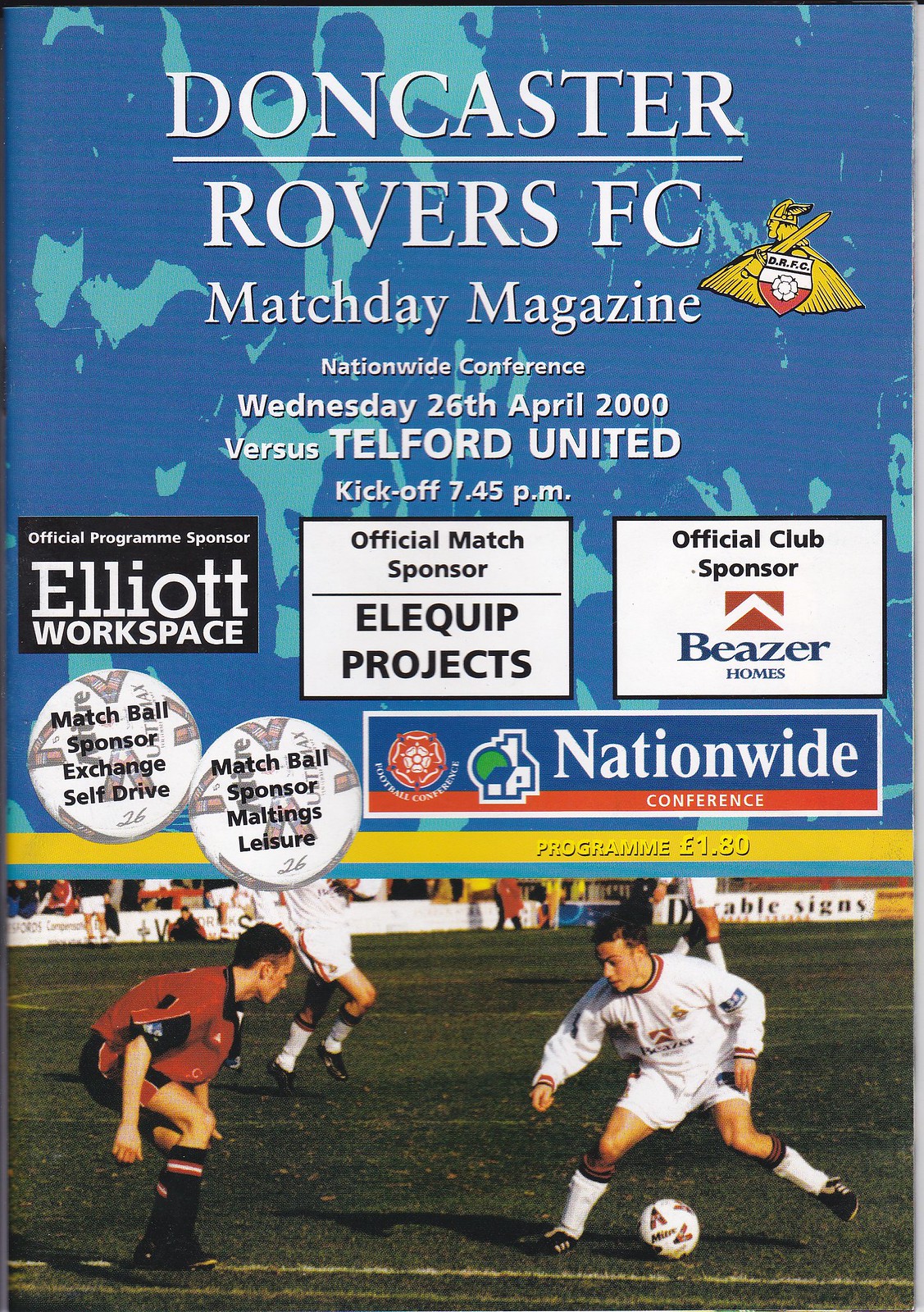The magazine cover for the Doncaster Rovers FC match day magazine features a dynamic blue background with light blue speckles at the top half, holding prominent white text that reads, "Doncaster Rovers FC Match Day Magazine." Below this, the yellow, red, and white Viking logo symbolizes the club's spirit. Further down is the announcement for the nationwide conference match against Telford United on Wednesday, April 26, 2000, with kickoff at 7:45 p.m. This information is accompanied by six logos representing various event sponsors, including "Elliott Workspace," "Allen Quip Projects," the official match sponsor in a white square, and "Beezer Homes," the official club sponsor, highlighted in diverse color fonts. The lower half showcases an action-packed soccer field scene where a player in white, controlling the ball, faces another in red and black gear to his left, with two additional players visible in the background. The imagery is underlined by a bold yellow bar stating "Program, £1.80."